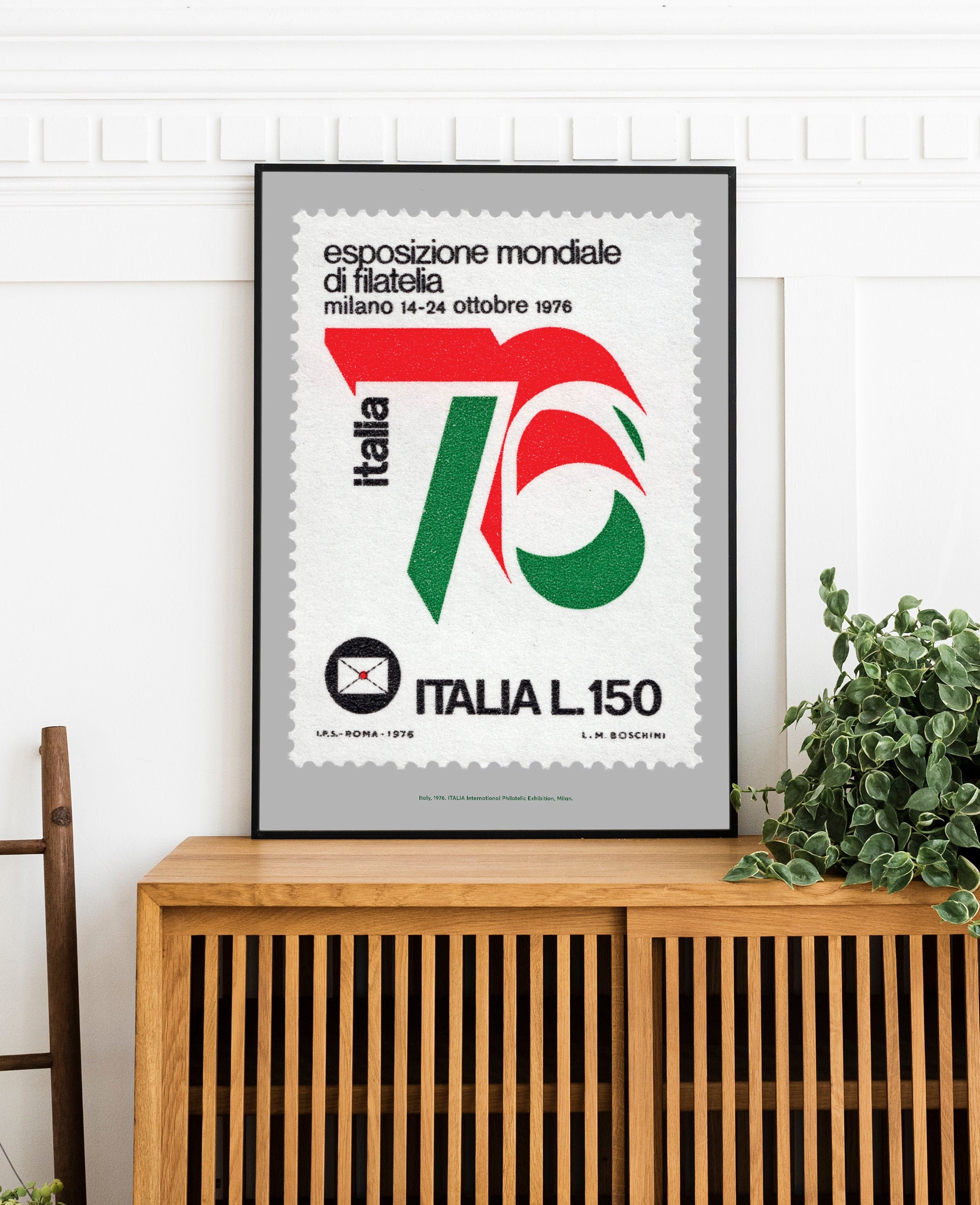In this photograph taken in an indoor setting, a light brown polished wooden cabinet with sliding doors and vertical slots is positioned against a white wall featuring square and rectangular patterns. Atop the cabinet sits a framed poster, propped upright against the wall. The frame is thin and black, and the poster resembles an enlarged postage stamp with serrated edges set against a grey background. The central part of the poster is white, displaying the text "Esposizion Mondial di Filatelia Milano 14-24 Octobre 1976" at the top, followed by a stylish number 70 in red and green hues, with "Italia L150" inscribed below. Notably, in the bottom left corner, "LPS Roma 1976" is printed, and in the bottom right corner, "LM Bosch Scenic" appears. Adjacent to the poster on the cabinet is a green potted plant with lush leaves. Additionally, to the side of the cabinet, there is a small wooden ladder.